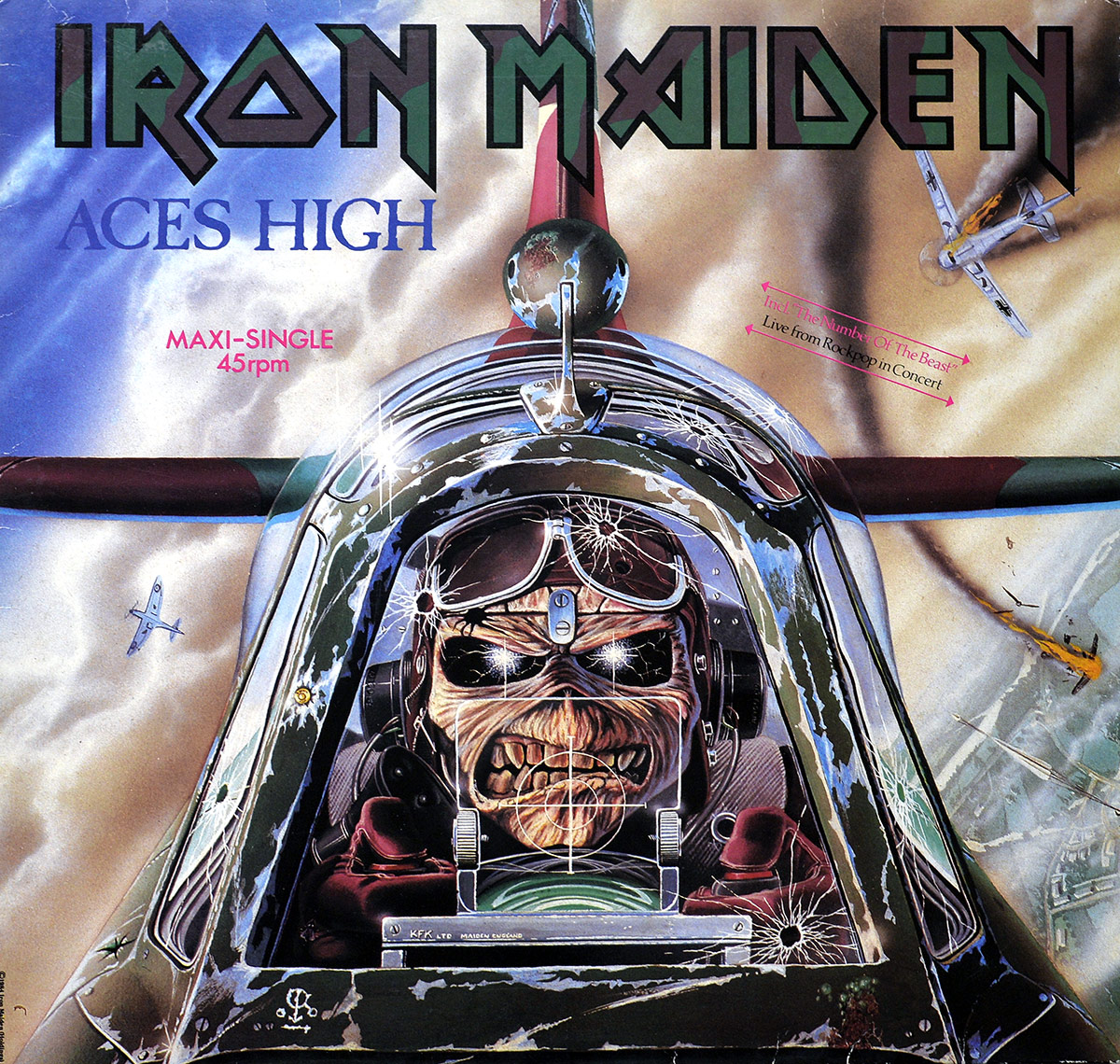The image is the cover of Iron Maiden's "Aces High" album, a maxi single 45 RPM vinyl, featuring the iconic dystopian warrior mascot, Eddie, depicted as a skeletal pilot. Eddie, with a face wrapped in tattered bandages and a grimacing mouth revealing jagged teeth, flies a black fighter plane with red and green details. His eyes, in the form of black voids with white lightning bolts, stare intensely out from under a battered helmet and goggles riddled with bullet holes. Wearing red gloves, Eddie has his fingers on the plane's triggers, guiding it through a chaotic sky where other planes are depicted crashing and ablaze. The cover is adorned with the words "Iron Maiden" in their traditional font camouflaged in green and brown, and "Aces High" along with "Maxi Single 45 RPM" and "Live from Rockpop in Concert" noted on different sections of the image. The scene is vividly set under a war-torn sky, enhancing the intense and haunting atmosphere of Eddie's airborne assault.